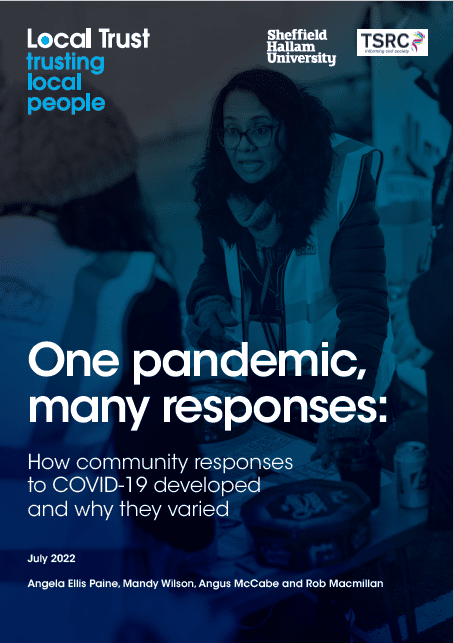The image is a vertically oriented graphic with a height roughly one and a half to two times its width. The background features a gradient blue color scheme, transitioning from a dark blue at the bottom to a medium blue in the middle, and finally to a lighter blue towards the top. The very top left corner uniquely shifts to a grayish hue. 

Overlaid onto this background is a scene depicting two women engaged in conversation across a table, positioned diagonally from approximately the 10 o'clock direction. The woman on the left, viewed from the back right-hand side, faces towards the upper right corner, while the woman on the right looks towards the lower left corner. The table holds some indistinct items, adding context to their interaction.

The overlay texts are positioned as follows:

- In the top left corner, the phrase "local trust" appears in white letters, with the "O" filled in with light blue.
- Below that, each word of the phrase "trusting local people" is placed on a separate line in light blue text.
- On the right-hand side, the text "Sheffield Harlem University" is present, alongside a logo reading "TSRC."
- Dominating the bottom half of the image is a large white text stating: "One pandemic, many responses. How community responses to COVID-19 developed and why they varied."

This detailed caption sets a clear and vibrant scene that conveys the essence and elements of the visual content effectively.